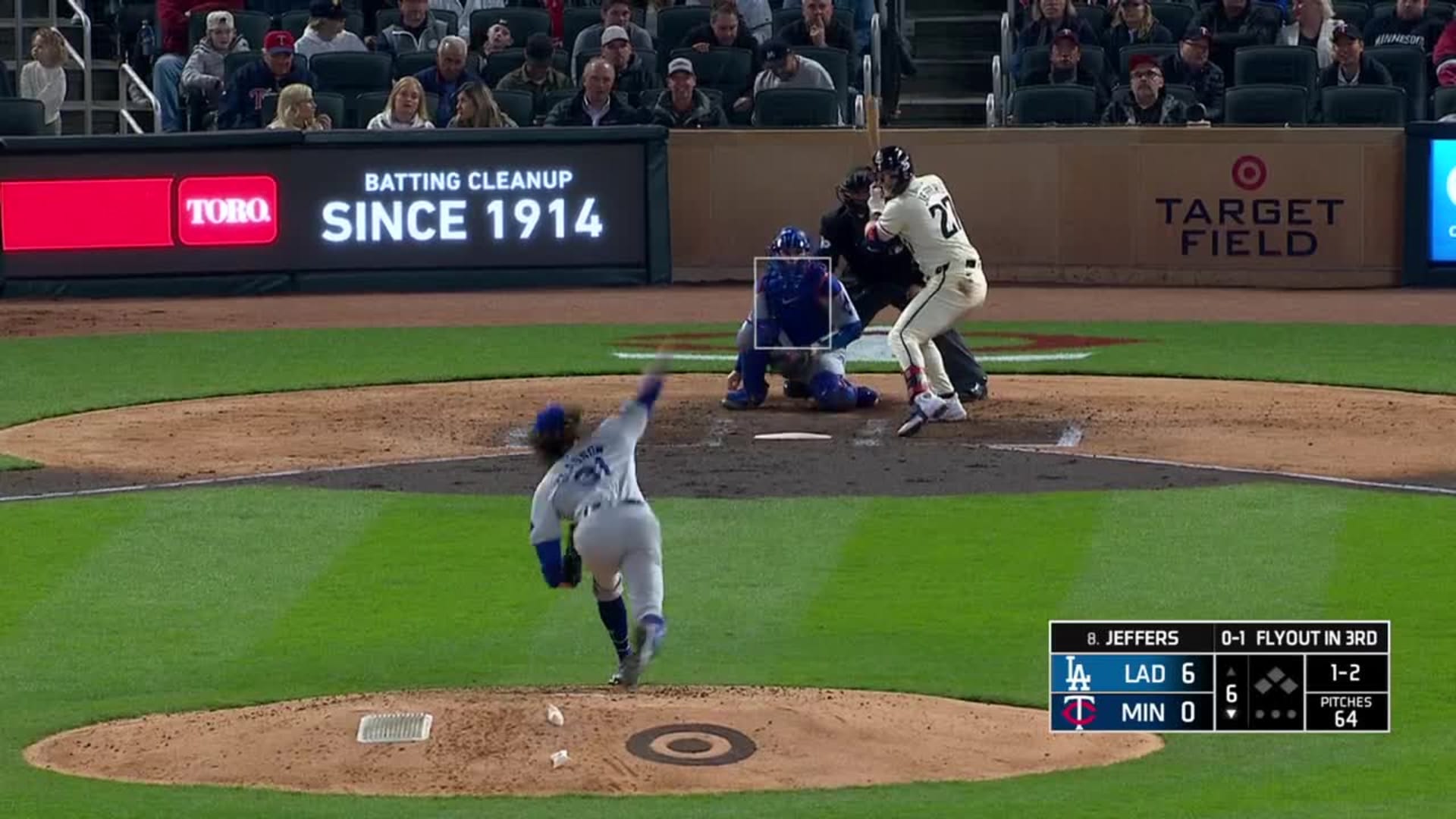The image captures a tense moment during a baseball game at Target Field in Minnesota. In the foreground, a right-handed pitcher in a blue and white uniform is poised to release the ball, while a right-handed batter, Ryan Jeffers, stands ready at the plate. Behind the batter, the umpire and catcher are positioned, completing the scene. The stands, not completely full, are visible in the background with fans seated in multiple rows. Various advertisements, including "Target" and "Toro Batting Cleanup Since 1914," adorn the stadium. The scoreboard indicates that it's the bottom of the sixth inning with the Los Angeles Dodgers (LAD) leading 6-0 against the Minnesota Twins (MIN). The count is 1-2, no runners are on base, and the pitcher has thrown 64 pitches. Jeffers is 0-for-1 with a flyout in the third inning. The Target logo is visible on the back of the pitcher's mound, reinforcing the game's location.